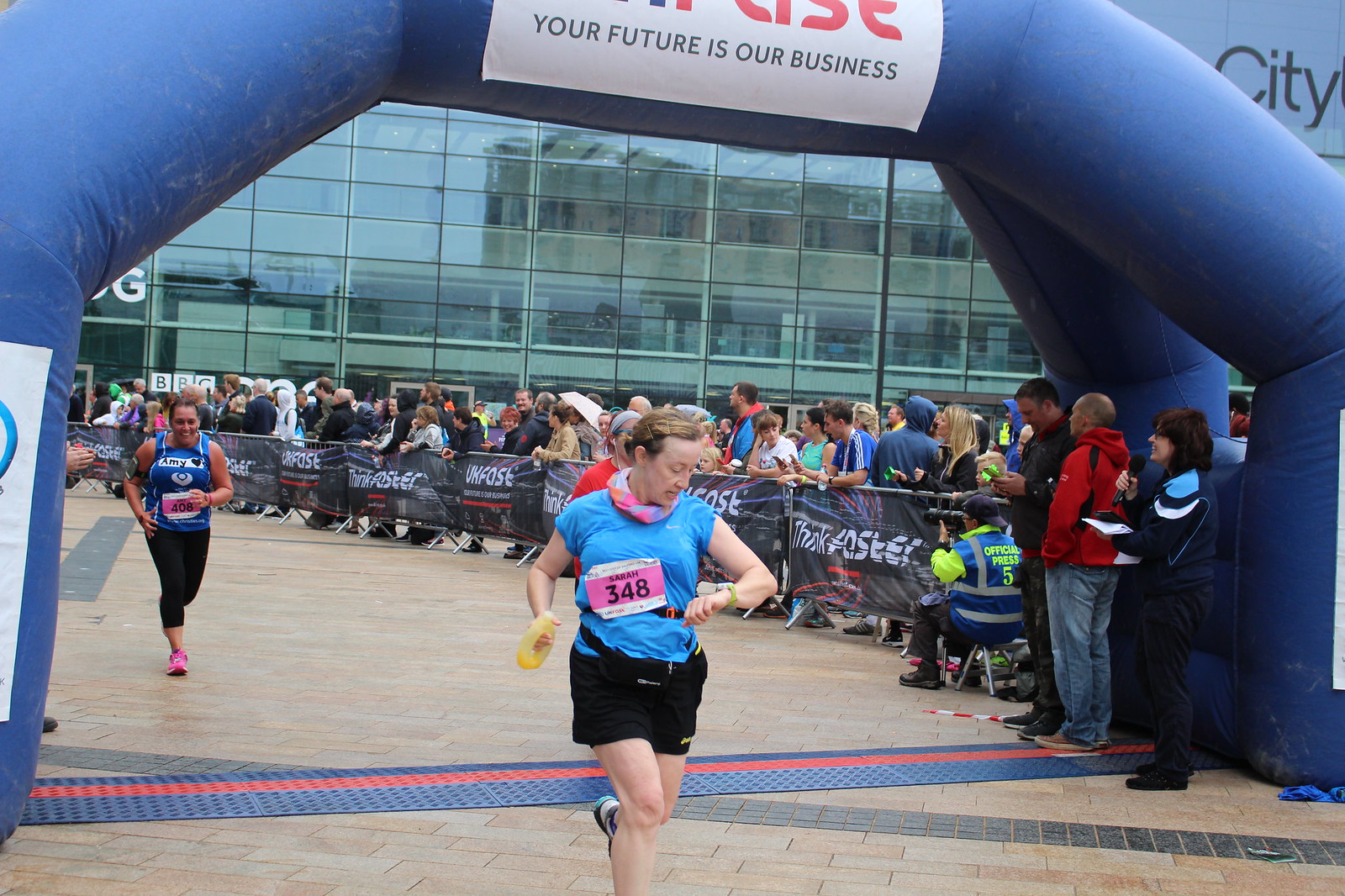In the image, an elderly white woman, estimated to be 45 to 50 years old, is crossing the finish line of what appears to be a marathon or a running event. She is wearing a blue shirt and black shorts, a bandana around her neck, and holding a yellow object, possibly a water bottle, in her hand. The woman, named Sarah, has her race number 348 pinned to the front of her shirt. She is looking at her watch as she completes the run. Behind Sarah is another woman, identified as Amy, who is wearing a blue tank top and similarly numbered with 408. Amy is wearing black capris and pink tennis shoes. Further behind them, there is a woman in a red shirt whose number is not visible. The race's finish line is marked by a large inflatable arch with the text "Your future is our business" displayed prominently. Spectators, around 30 in number, are lined along a fence, watching the race near a modern glass building marked with "BBC," indicating it's possibly a television and radio station. Several officials in blue coats can be seen monitoring the event.